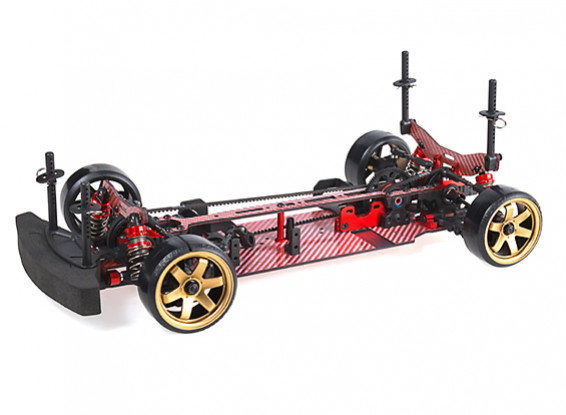The image depicts the incomplete chassis of an RC car, displayed on a white background. This partially constructed toy car highlights its intricate internal mechanics and lacks an exterior frame, emphasizing its unfinished state. The undercarriage is adorned with a striking red and white stripe pattern, while the wheels are black with prominent gold-plated, six-spoke rims. The visible mechanical components, composed of various metals and plastics, include springs and a central bar that stabilizes the structure. At the front and rear, two poles project upwards, with the rear set slightly taller, possibly intended for mounting additional parts or accessories. A small black plastic bumper is attached at the front, and another black bumper is visible at the back. The overall view showcases the RC car’s inner workings, hinting at its potential once fully assembled.